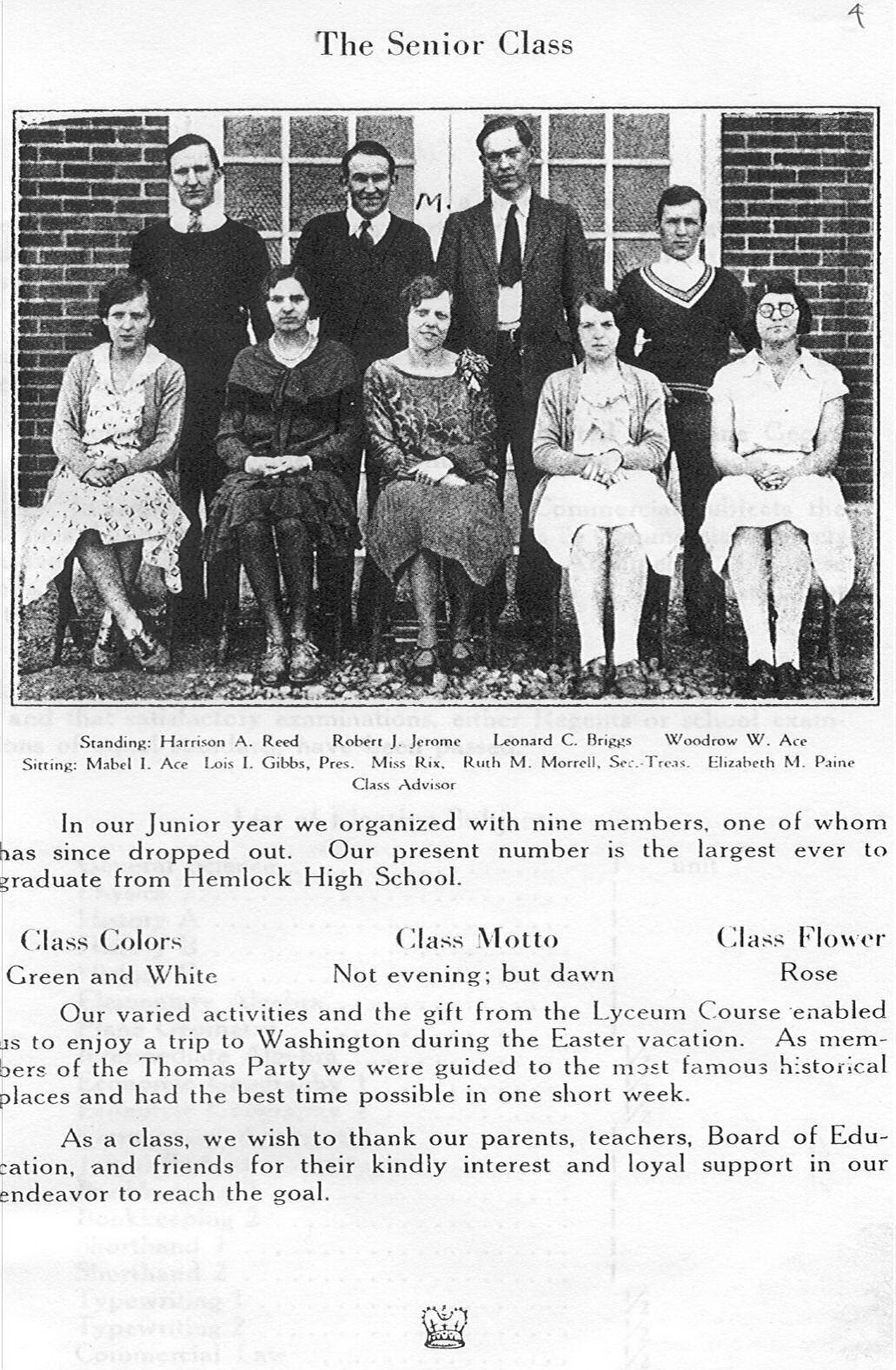In this vintage, black and white class yearbook photo titled "The Senior Class," nine formally dressed individuals pose in two rows against a brick building with white windows and doors. The top row features four men: Harrison A. Reed, Robert J. Jerome, Leonard C. Briggs, and Woodrow W. Ace. The outer men wear sweaters, the left in a crew sweater and the right in a V-neck, while the central two don suits with dark ties. The bottom row presents five women seated: Mabel I. Ace in a white and dark print dress, Lois I. Gibbs in a dark dress, Miss Riggs in another dark dress, Ruth M. Morwell, the secretary, in a white dress with a sweater, and Elizabeth M. Payne, the class advisor, in a white dress. The accompanying text reminisces about organizing as juniors with nine members, one of whom has since dropped out, and proudly mentions their class as the largest ever to graduate from Hemlock High School. Their class colors are green and white, the motto "Not evening but dawn," and the class flower is the rose. Reflecting on their collective experiences, they recall a memorable Easter vacation trip to Washington, funded by the Lyceum course, where they explored significant historical sites as part of the Thomas party. The students express gratitude towards their parents, teachers, Board of Education, and friends for their support in reaching their academic goals. The page also features a drawing of a crown at the bottom center.